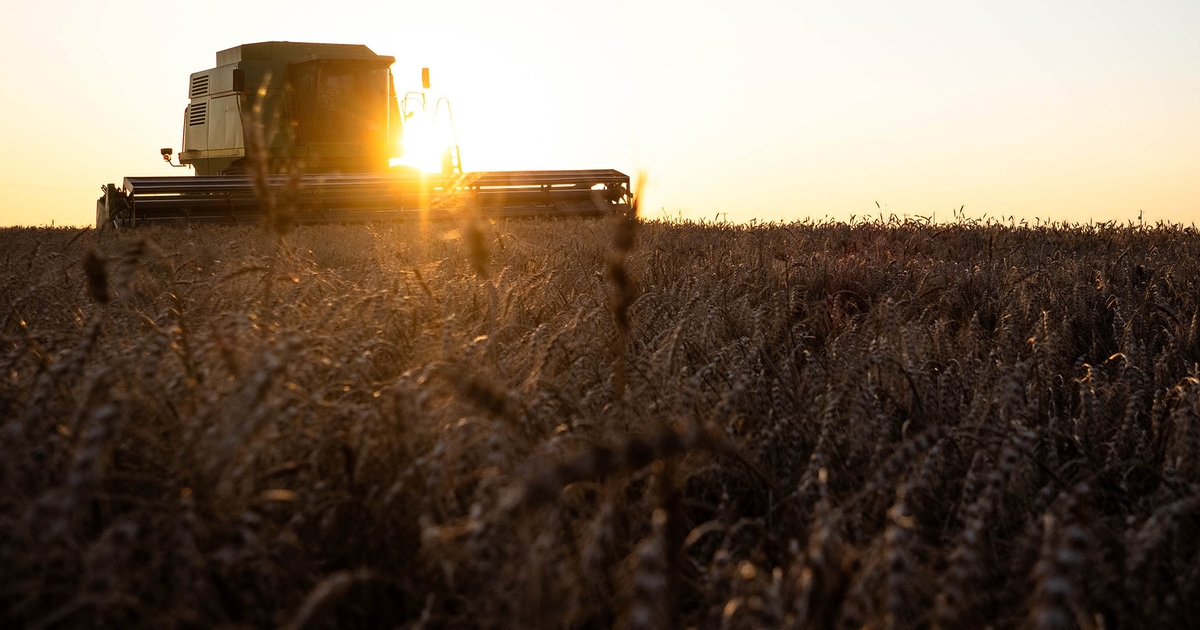Captured in the soft light of either early morning or dusk, this professional artistic photograph beautifully depicts a vast, golden wheat field stretching endlessly into the horizon. The sky above transitions from a light blue at the top to a warm orange closer to the horizon, with the sun low in the sky casting a gentle glow across the scene. In the top left corner of the image, bathed in the sun’s radiant bloom, stands a large, yellow combine harvester. This boxy vehicle features a prominent windshield and a sizable, rectangular rotating mechanism at its front, poised for harvesting the ripened wheat. The sunlight partially obscures the finer details of the harvester, creating a bright halo effect around it. The wheat field itself is densely filled with stalks, their golden hues suggesting they are ready for harvest. Despite the focus on the harvester, the image's depth of field also allows for a detailed, yet slightly blurred view of the individual wheat strands in the foreground, emphasizing the rich texture and abundance of the field.